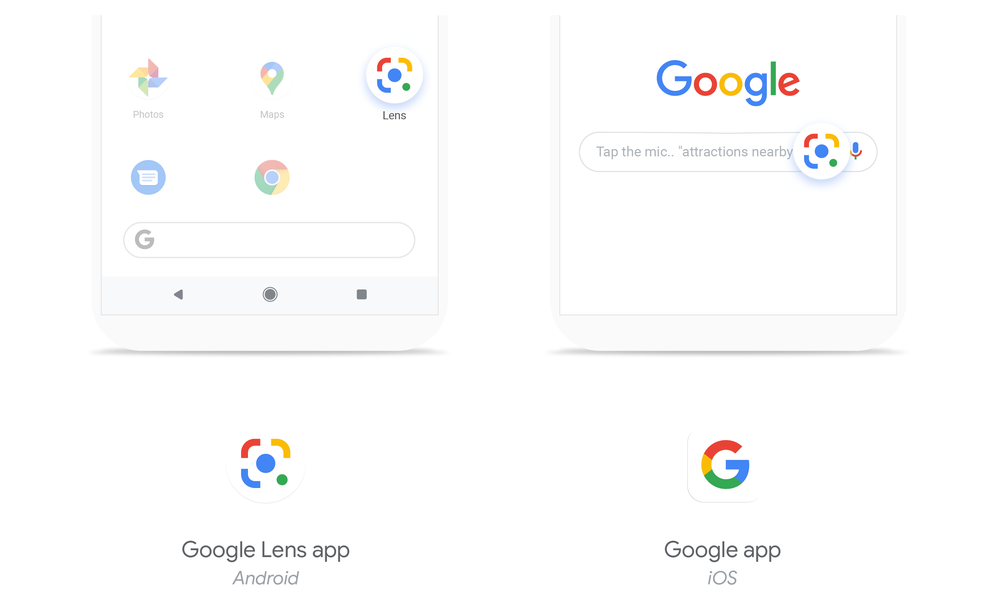The digital image prominently features the Google logo, which consists of a capital 'G' in blue, followed by a lowercase 'o' in red, another lowercase 'o' in yellow, a lowercase 'g' in blue, a lowercase 'l' in green, and a lowercase 'e' in red. Below the logo, there is a search bar with the text "Tap the mic, attractions nearby," accompanied by a microphone icon in blue, red, yellow, and green colors. To the left side of the image, there are icons for several Google-related apps: Photos, Maps, Lens, Google Chrome, and another Google search bar. Additionally, the image shows the Google Lens app for Android and the Google Maps app for iOS.